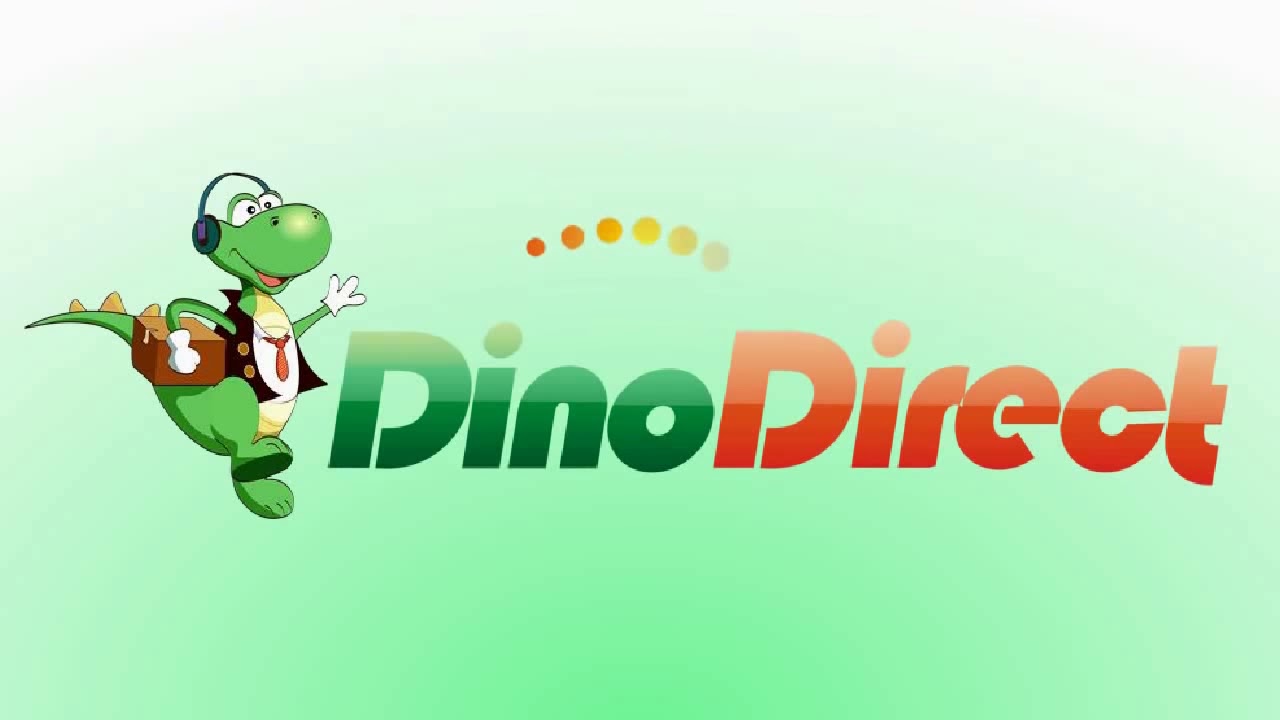The image showcases a company logo set against a light green background that fades to white at the top edges. Centrally positioned is the text "DinoDirect," with "Dino" in green and "Direct" in red. To the left of the text stands a detailed, cartoonish dinosaur. The green dinosaur has a yellow and white chest, orange scales on its tail, and is adorned with black headphones. It is dressed in a white collared shirt, red tie, white gloves, and a black jacket with brass buttons. The dinosaur stands upright on its hind legs, smiling as if dancing or skipping, and carries a brown wooden chest securely under its right arm. Above the text, a series of six circles transition in size and color from smaller, darker orange on the left to larger, brighter yellow and white on the right. The layout and detailed design suggest it could be an advertisement or a logo suited for a business card.